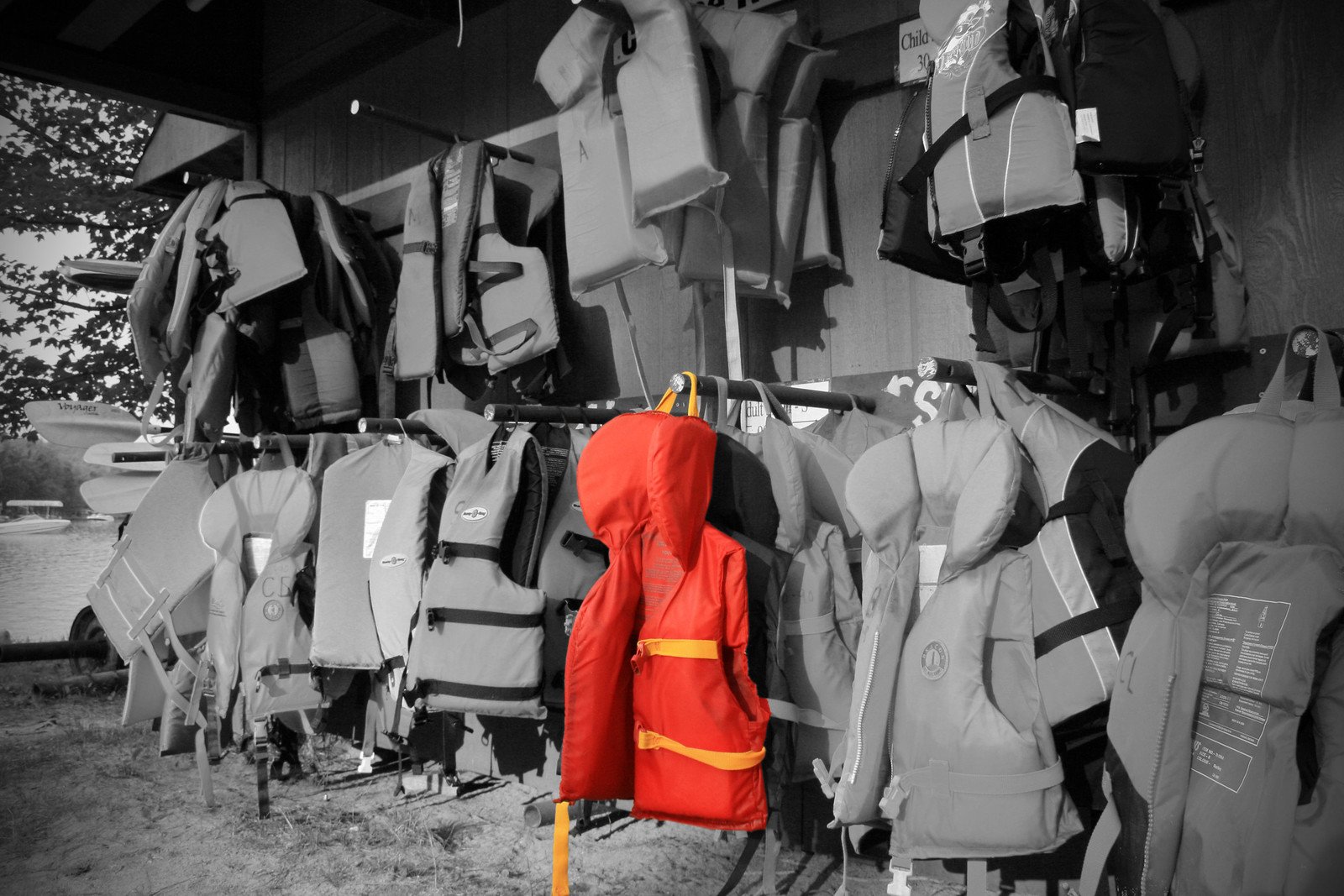The black and white photograph captures the rustic essence of an outdoor boathouse, identifiable by its long, two-story brown wood-paneled wall. The wall is covered with rows of life jackets hanging from metal poles, arranged in sizes suitable for both children and adults. The image's focal point is a vibrant orange life jacket with yellow straps, conspicuously colorized amidst the grayscale setting, positioned on the fifth hook from the left on the bottom row. In the background, beyond the boathouse, lie serene waters dotted with a couple of distant boats, likely in a lake or pond, and flanked by trees with thin branches and full foliage. The dark shades of a nearby roof under an overhang also add depth to the photo, highlighting the boathouse’s utilitarian purpose.